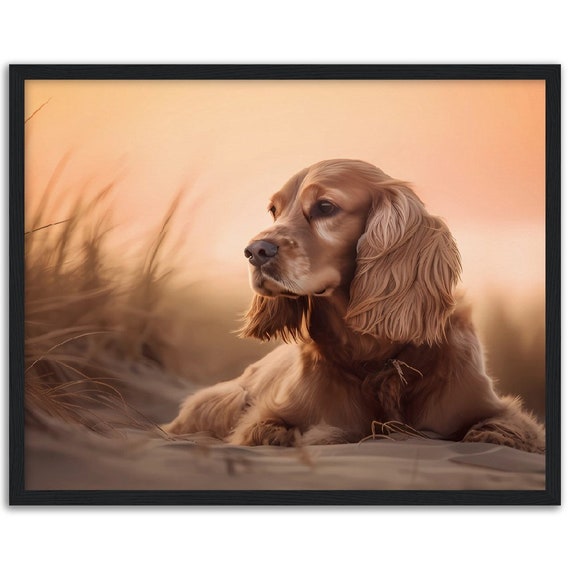This color photograph, possibly AI-generated or edited, features a dog that resembles a Golden Retriever or a Cocker Spaniel with distinctive long, shaggy, reddish-brown ears. The dog has a reddish-brown coat with a lighter, almost white snout and lighter patches under its eyes. It sits on fine, light brown sand on what appears to be a beach, with its head looking slightly to the left and the rest of its body out of view. To the left of the dog, there is tall, brown seagrass, while more grass fades into the out-of-focus background. Overhead, the sky showcases a serene sunset with hues of pink, orange, and yellow clouds. The entire image is encased in a thin black frame, presenting a tranquil and possibly artificial or computer-generated seaside scene.